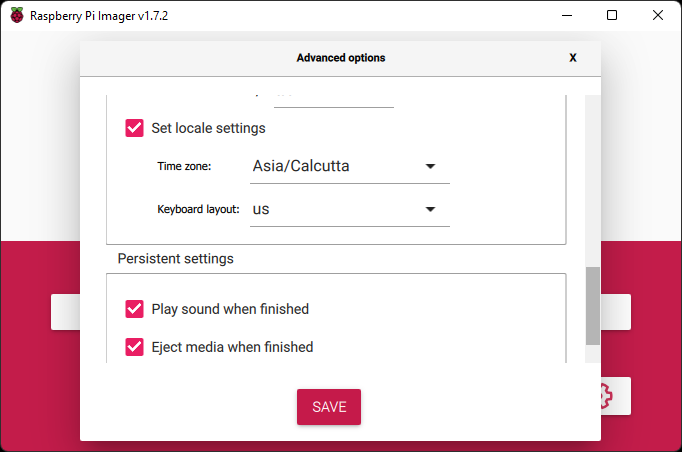This is a detailed, descriptive caption for the image:

---

The screenshot features the Raspberry Pi Imager interface. In the top-left corner, the Raspberry Pi logo is prominently displayed, alongside the text "Raspberry Pi Imager v1.7.2." On the right-hand side, there are three familiar window control icons: a minimize icon (represented by a dash), a maximize icon (a square), and a close icon (an X).

Below, centrally aligned at the top, is a large square section labeled "Advanced Options." In its top right corner, there is an "X" icon for closing the window. Within this section, the first item is a pink box with a white checkmark, next to the text "Set Locale Settings." 

Following this, there is a line labeled "Time Zone," with a dropdown menu set to "Asia/Calcutta." Below this, another line is labeled "Keyboard Layout," with a dropdown menu set to "US."

Further down, there's a box labeled "Persistent Settings." Inside this box:
- A pink box with a white checkmark next to "Play Sound When Finished."
- Below it, another pink box with a white checkmark labeled "Eject Media When Finished."

At the very bottom of the "Advanced Options" section, a centered, rectangular red button labeled "Save" is prominently displayed.

The entire Advanced Options section is superimposed upon the Raspberry Pi Imager interface. The background behind this section is minimal, with the top half white and the bottom half dark pink. Some additional boxes are partly visible in this background, though their contents are not clear.